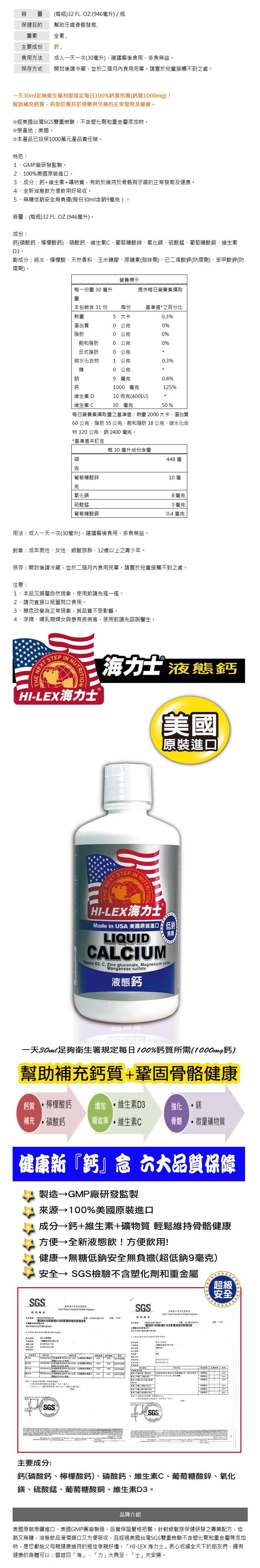The image is a detailed, vertically long series of labels that appear to be for a liquid calcium supplement. At the top, the background is primarily white with extensive black text and a couple of lines in red font. This section resembles nutritional or supplement facts, structured in a table layout. Below, a white plastic bottle with a screw top features prominently. The label on the bottle reads "Liquid Calcium" in black letters against a greyish background, with a distinctive blue banner piece at the bottom. The top portion of the label has legible text, but the details are difficult to decipher. Adjacent to the bottle is a red, round logo, possibly representing a globe, overlaying an American flag, which has a blue background with white stars, and red and white stripes. Further down the image, there's a series of colored symbols and arrows, including a yellow circle with white pox, red, green, and purple arrows pointing at various ovals, and blue Chinese characters. The bottom part includes a mix of bolded black text and more nutritional information in a red-outlined box. Some sections are particularly small and hard to read, emphasizing that the label contains multilingual elements, likely in English and Chinese.